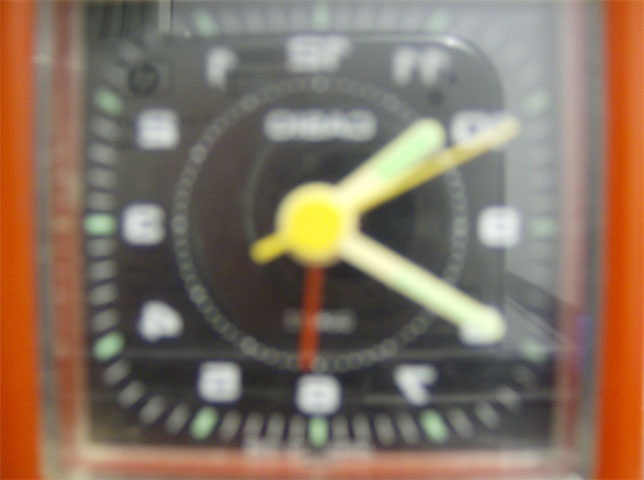The image depicts a very blurry, squared clock or gauge with a red frame, viewed from an overhead perspective and encased in a plastic or glass casing. The face of the clock appears black with white numbers 1 through 12, though they are difficult to discern clearly due to the blurriness and some numbers appearing reversed. The clock features white and green marks—green ticks mark each number with four smaller white ticks between them. Inside the main numeric scale is another, indistinct scale with light green and yellow colors. The clock has three hands—one yellow second hand pointing to the two o'clock position, a white hour hand at ten, and a white minute hand at eight. Additionally, there’s a smaller, yellow mini dial at the bottom pointing to eight, possibly for micro-seconds. The surrounding background color is orange, adding to the overall vibrant but confusing appearance of the image.